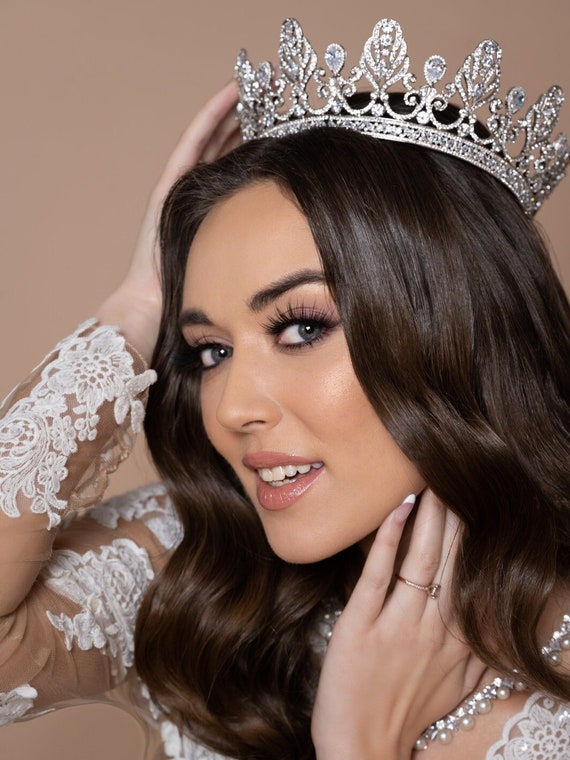The image features a close-up of a beautiful Caucasian bride against a solid light brown background. Her makeup is impeccably done, with foundation, curved dark eyebrows, and possibly artificial long black eyelashes highlighting her striking blue eyes. She has shiny, wavy brown hair cascading over her shoulders and wears a floral, lacy gown with semi-transparent sleeves. 

The bride is adorned with an elegant silver tiara encrusted with diamonds, which she is touching gently with her right hand, bending her elbow to do so. Her left hand rests gracefully with fingertips touching the side of her chin. Around her neck, she wears a sophisticated necklace that combines pearls and diamonds. She is smiling slightly, revealing her teeth, and has applied a rosy pink lipstick to her lips.

In the lower right part of the image, the intricately designed top of her gown is visible, further accentuating her elegant appearance. The overall composition of the picture is highly aligned, capturing the essence and grace of the moment.